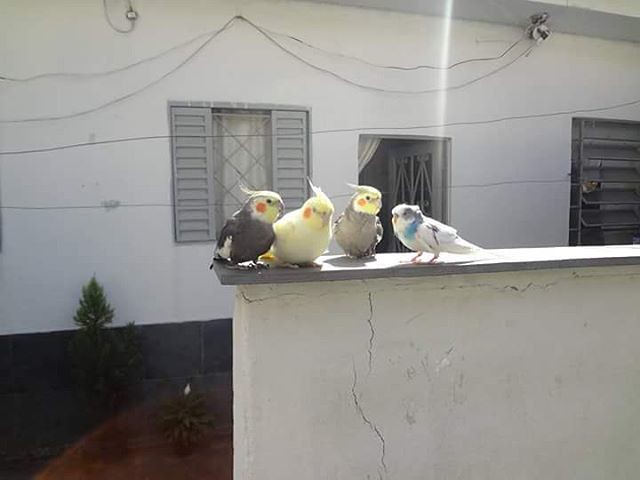This outdoor photograph captures a bright, sunlit scene featuring four distinctively colorful birds perched on a cracked, white cement wall with a narrow grey ledge. Three of these birds are cockatiels: one is primarily grey with a yellow face and bright orange cheeks, another is mostly yellow with similar facial markings, and the third is lighter grey with the characteristic yellow and orange cheek patches. The fourth bird, distinct from the cockatiels, is a white-breasted parakeet with a blue patch on its neck. The background reveals a slightly run-down white house with grey shutters and an open door. The exterior of the house is adorned with multiple power and CCTV cables, and there's a small bush situated at the bottom left side of one of the windows. The house and the perched birds are bathed in sunlight streaming from the top right, creating a vibrant and detailed composition.